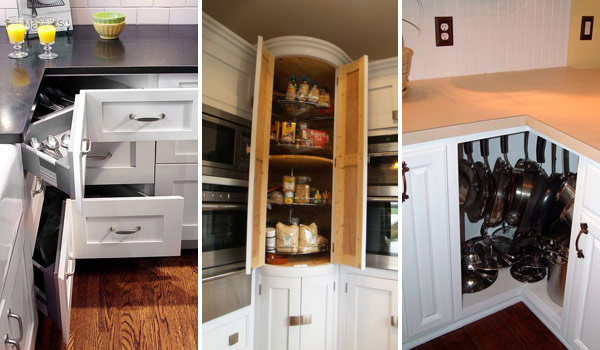This image displays three vertically aligned photographs, each capturing a unique kitchen storage solution focused on corner utilization. 

In the left photograph, the scene features a white kitchen with black quartz countertops. A set of intriguing triangular drawers are pulled open, showcasing brushed nickel handles and containing silverware. The countertop holds two small glasses of orange juice and an olive green bowl stacked on a beige one. The kitchen's floor is dark wood plank, and a white brick wall adds texture in the background.

The middle photograph presents another white kitchen cabinet, this time a corner unit equipped with a four-tier Lazy Susan. The rotating shelves are stocked with various food items. Notably, this cabinet is positioned next to four ovens, enhancing its functional appeal.

The right photograph illustrates a corner cabinet with a salmony cream-colored countertop beneath. White cabinets with hanging pots add to the organized look, offering a practical storage solution for cooking utensils. 

Together, these images provide a comprehensive view of innovative ways to optimize corner space in a kitchen.